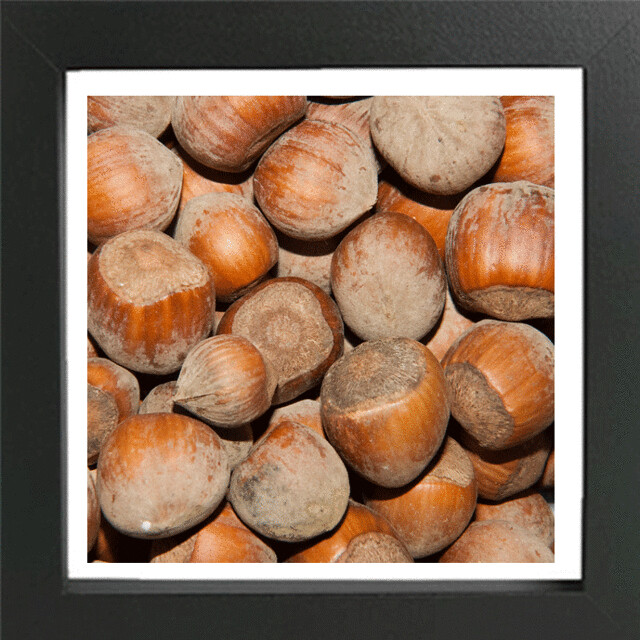This is a detailed product photo featuring a close-up image of various nuts, potentially chestnuts, filberts, or pecans, with their original shells. The framed photo is encased in a solid black frame with mitered corners and includes a white matting that creates a narrow, contrasting border around the main image. The nuts, which range in shades from medium brown to a golden brown, are piled together and exhibit vertical striations on their sides. Many of the nuts have flat, rough tops, while their bottoms vary from pointed to rounded shapes. One notably smaller nut sits atop the pile with a distinctly pointier bottom. The nuts appear to be dirty or dusty, featuring light brown dirt and dried particles on their surfaces, and there are some light reflections highlighting their textures. The framed image has no text or additional information, keeping the focus entirely on the natural, uncleaned state of the nuts.